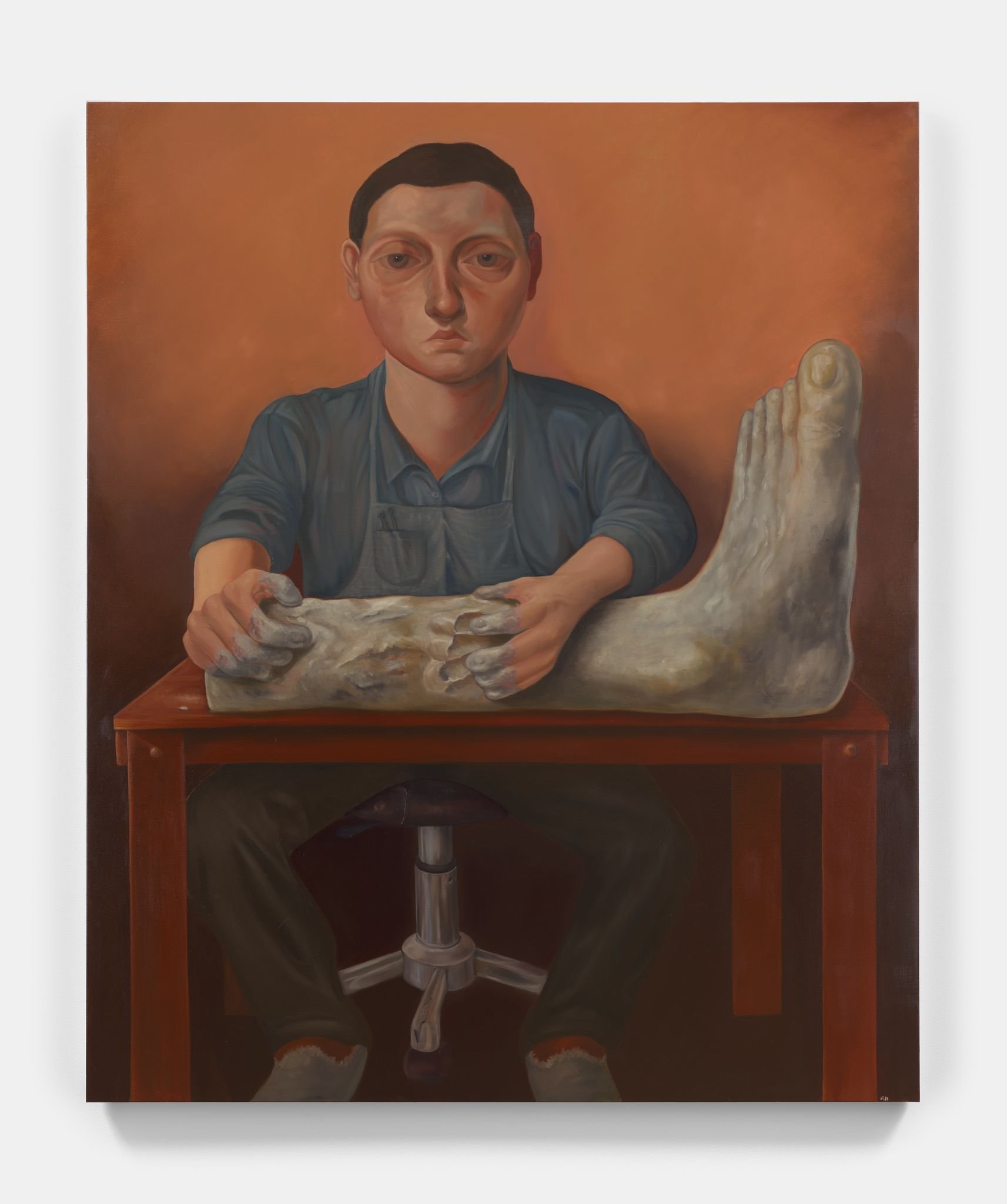The painting depicts a solemn, stylized man with an exaggerated, cartoonish appearance located against a brown, muddy background. The figure, a white male with large, expressive eyes and disproportionately small body relative to his large neck and head, sits on a swivel office chair with a spring mechanism for height adjustment. He is dressed in a blue shirt with rolled-up sleeves, complemented by a matching full-length apron. The man intently works with clay, shaping a misshapen, oversized leg on a rustic wooden red table in front of him. His large hands, smeared with clay residue, and visible fingerprints in the wet clay suggest a hands-on creative process. The man’s short brown hair, long nose, and stoic, serious expression, as he gazes directly at the viewer, add an emotional depth to the folk-art style painting.